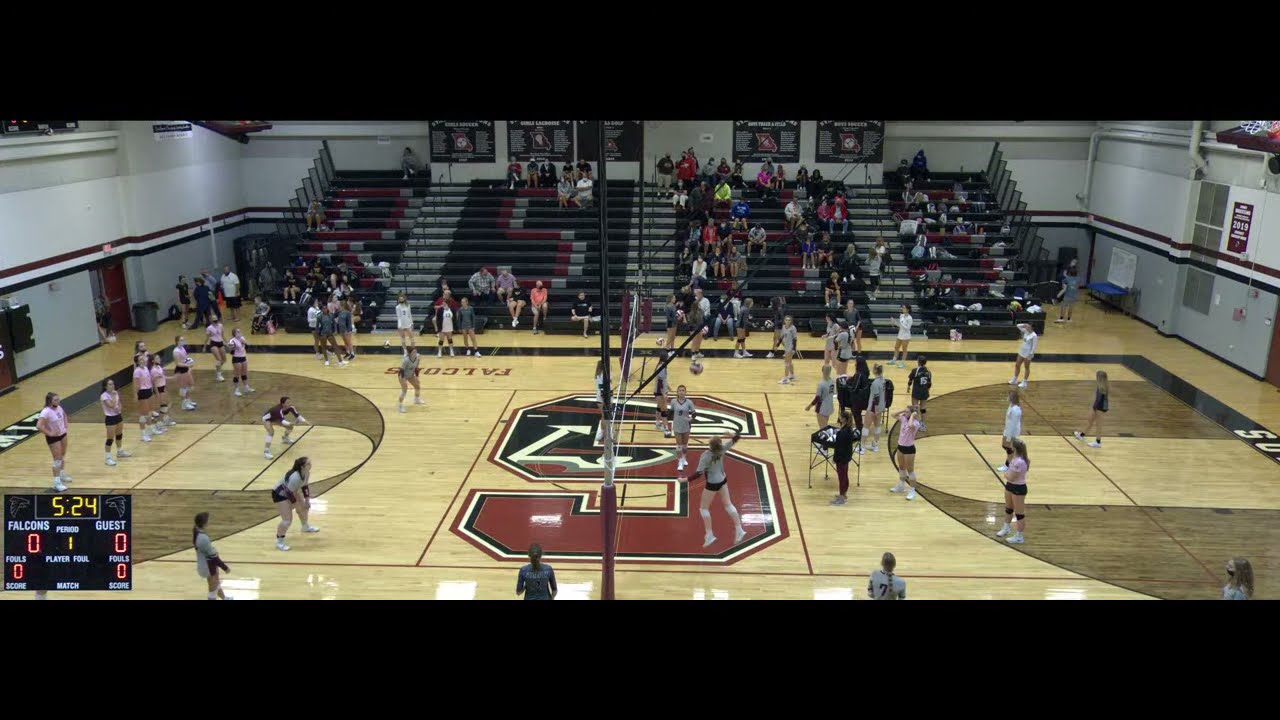This indoor image captures a volleyball game in a gymnasium, most likely during a warm-up session. The court, marked with a large red and black "S" in the center, features the logo of the home team, the Falcons. Players, coaches, and staff are scattered across the court, which is composed of various shades of brown. The team uniforms include pink jerseys with black shorts and white shoes, as well as gray jerseys with black shorts and white shoes. 

In the bottom left corner is a scoreboard showing the competitors—Falcons and Guests—both with scores of zero, and a timer indicating 5 minutes and 24 seconds remaining. The scoreboard also displays fields for period, player foul, match, and fouls. The gymnasium's walls are gray with red and white stripes, adorned with pennants and flags. 

At the top of the image are bleachers populated by fans, whose attire includes striking colors such as lime green, blue, and salmon. Above the bleachers, signs and banners are visible, enhancing the vibrant atmosphere of this sports event. The gym's high walls are painted white with red and black trim, adding to the structured yet lively ambiance of the venue.